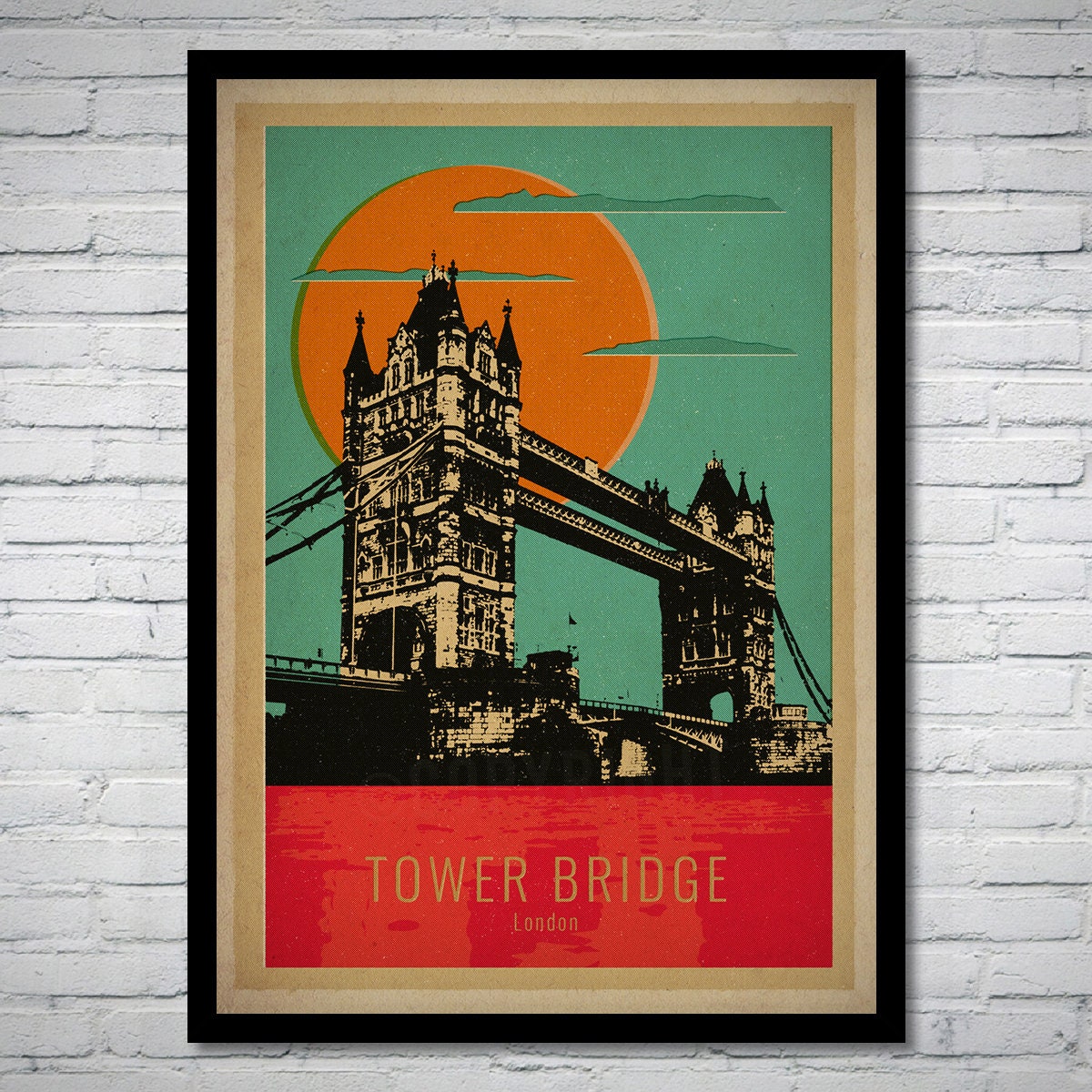This photograph captures an art piece hanging on a white brick wall. The framed artwork, which features black, light beige, and darker beige elements, vividly portrays the Tower Bridge in London. The majority of the piece is a black and white drawing of the bridge from a perspective as if seen from sea level, looking upwards. The backdrop includes a striking blue sky with several teal-colored clouds and a perfectly circular, large orange sun behind the bridge. Below the drawing, a bold red rectangle contains the inscription "Tower Bridge" in big yellow letters and "London" in smaller font. The artwork also bears a faintly visible watermark. The frame is a blend of black with layered light brown and gray accents.